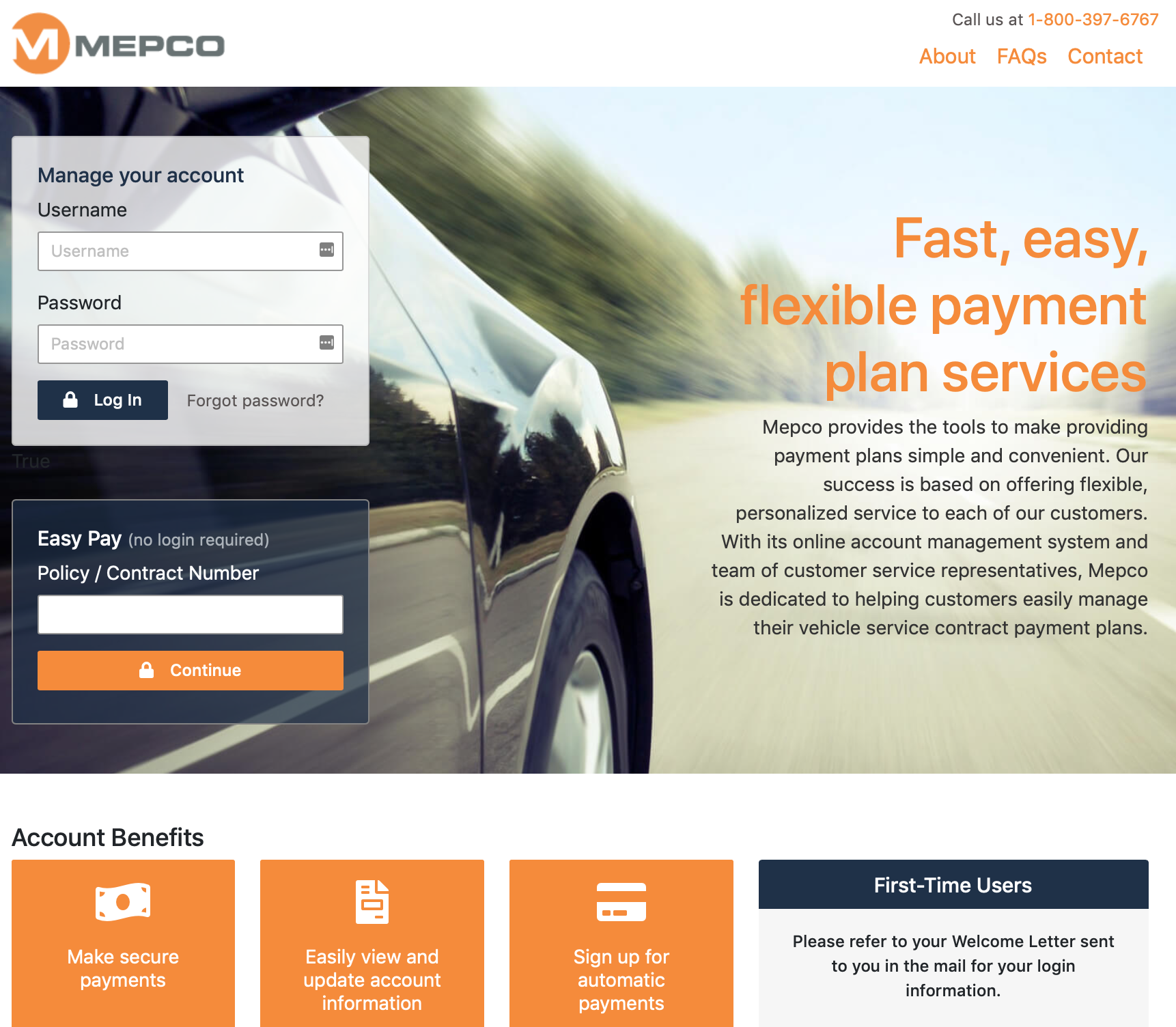In the image, a website interface for making car payments is prominently displayed. At the top of the page, the company name "M-PICO" (spelled M-E-P-C-O) is featured alongside their distinct "M" logo. Below this header, a large background image of a moving car sets the dynamic tone of the page.

Overlaid on the right side of this car image is a gray box labeled "Manage Your Account." Here, users can input their username and password, with options for login and retrieving forgotten items.

Adjacent to the gray box, there's a blue box titled "Easy Pay - No Login Required," where users can enter their policy and contract number before pressing "Continue."

On top of the car image, bold orange text reads "Fast, Easy, Flexible Payment Plan Services," accompanied by a brief description of the M-PICO company.

Beneath the large image, four feature boxes further detail the site's functionalities under the header "Account Benefits." The first three boxes are orange:
1. "Make Secure Payments" with a dollar icon.
2. "Easily View and Update Account Information" with a paper icon.
3. "Sign Up for Automatic Payments" with a card icon.

The fourth box stands out with a blue header and gray background. It is directed towards first-time users, advising them to "Refer to your welcome letter sent to you in the mail for your login information."